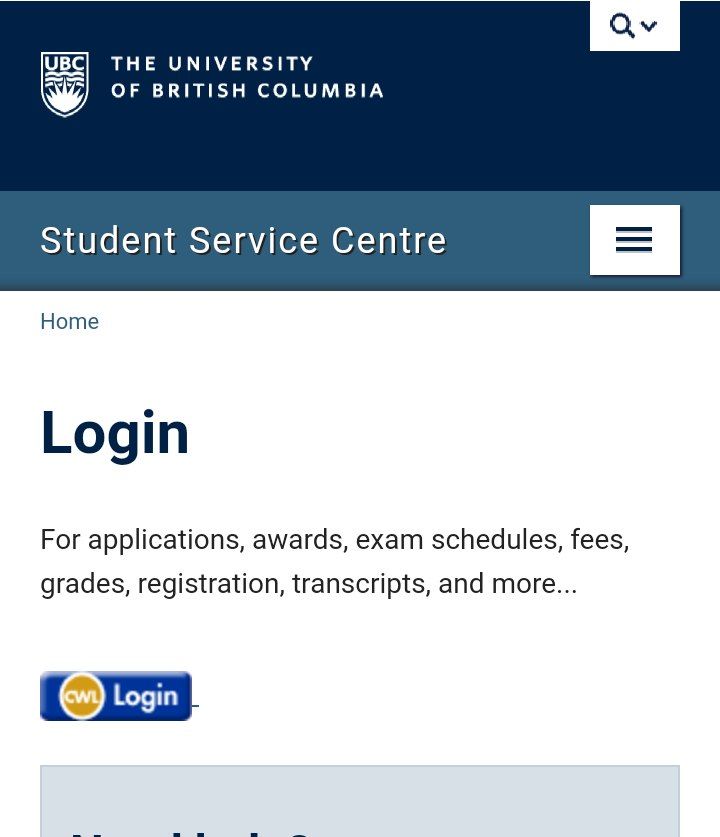Screenshot from the mobile site of The University of British Columbia:

The screenshot captures the top third of the page. At the very top is a wide navy blue border with white, capitalized fonts. On the left side, it reads "The University of British Columbia," and beside it to the left is the university seal. The seal is also white and includes the letters "UBC," wavy horizontal lines, and a drawing of a sun at the bottom, all enclosed in an inverted dome shape.

On the upper right corner, a square shape houses a search icon—a circle with a line extending to the lower right—and an inverted arrow, denoting a search drop-down box. Below this section, the color shifts to a light grayish blue. Here, a narrow rectangle spans left to right with the text "Student Service Center" in white font. On the right side of this rectangle, a white square containing three horizontal lines indicates a drop-down menu.

The background below this section turns white. On the left side, in very small letters, it says "home." Below this, in large black font, it reads "Log in." Underneath, in regular-sized, non-bold text, it lists, "for applications, awards, exam schedules, fees, grades, registration, transcripts, and more."

Further below, there is a royal blue rectangle with "Log in" written in white. Additionally, there is a gold circle outlined in white, featuring the letters "CWL."